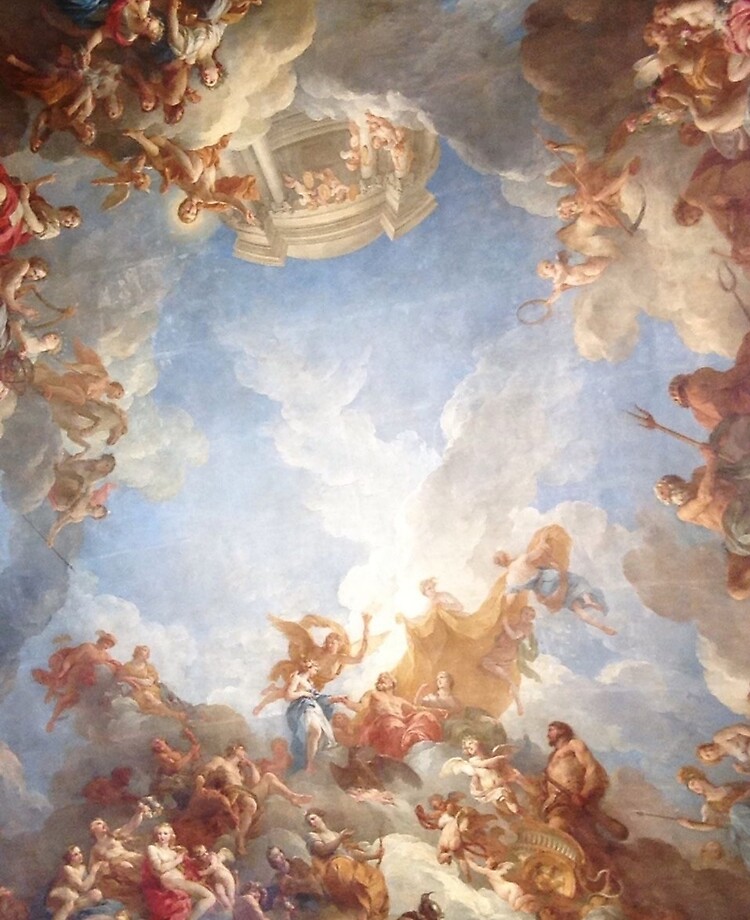The image appears to be a highly detailed and possibly medieval-inspired painting that evokes the ethereal quality of a dream. Dominating the scene are numerous angelic figures with wings, floating gracefully in the air. The humans, clad in flowing garments, engage in various actions—some are locked in battle, with detailed depictions of men clashing with pitchforks or spears, while others, primarily women, seem to be pulling warriors away from the fray. The central focus is a radiant, bright light that illuminates the sky, adding a heavenly glow to the scene. This celestial light seems to be viewed from the ground, drawing the observer’s eyes upwards. The sky's backdrop is a blend of light blue and soft clouds, dividing the dynamic war scenes that border the composition. Scattered around the edges are people in hues of brown and red, communing and gazing at each other, evoking a sense of otherworldly calm amidst the chaos. The overall aesthetic bears a resemblance to the intricate ceiling art found in places like the Vatican, yet it introduces a unique medieval feel with a panoramic spread of figures and dramatic action.